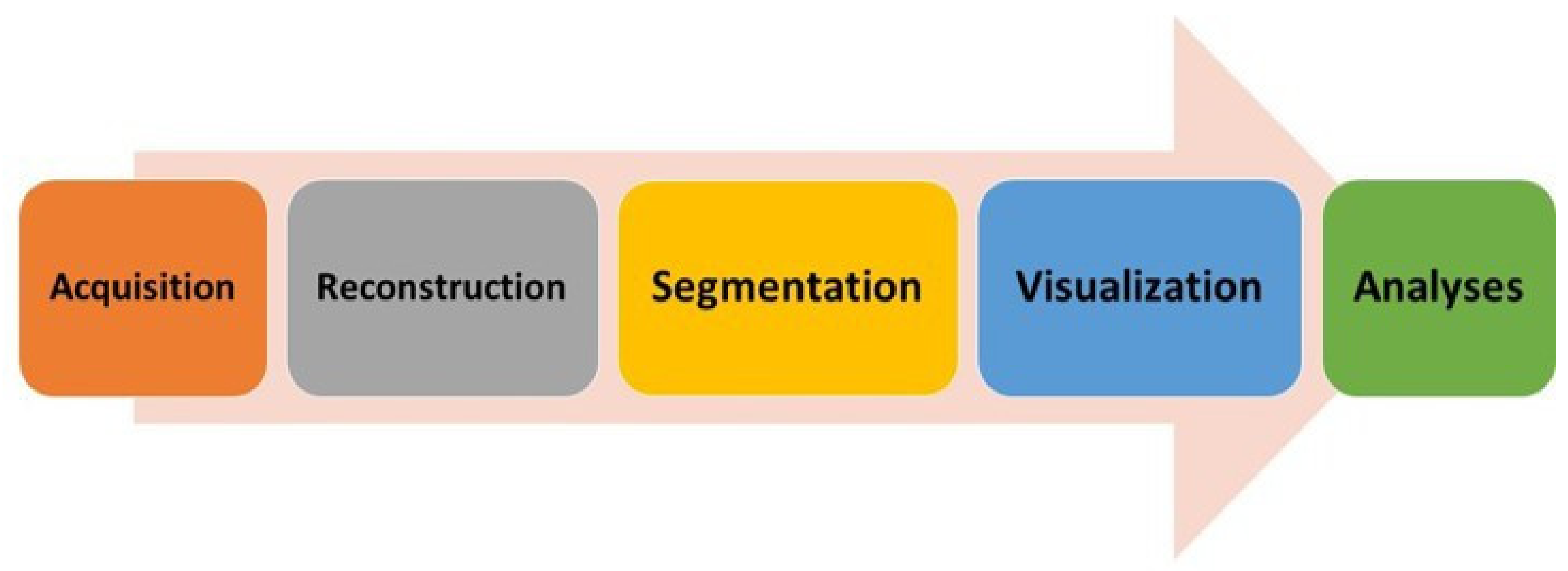The image is a detailed graphical representation of a five-step process, depicted through a flow chart with a large beige arrow pointing from left to right on a white background. This arrow indicates the direction of progression, starting from the left with the term "acquisition" in an orange rectangle. Following this are "reconstruction" in a slightly larger gray rectangle, "segmentation" in a yellow rectangle, "visualization" in a blue rectangle, and finally, "analysis" in a green rectangle at the arrow's pointed tip. Each rectangle, which contains the respective step's title, has rounded corners, contrasting with the sharpness of the arrow. This illustration appears to be a structured visual guide, possibly from a textbook, summarizing the sequential stages of a given process.